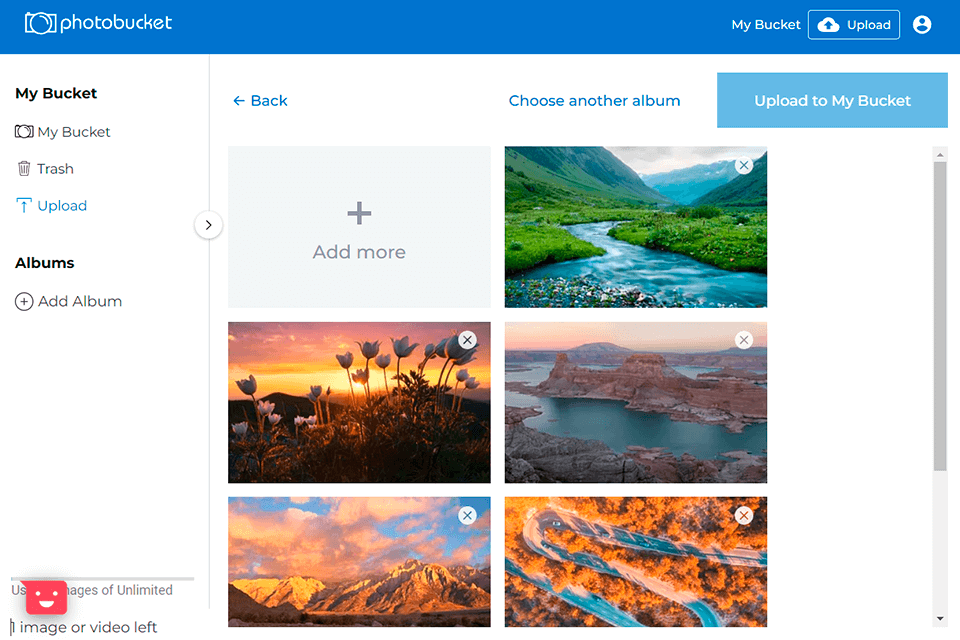This image captures a computer screen displaying the interface of the Photobucket website.

At the top of the screen, a blue background features the Photobucket logo in white text on the left side, along with an icon of a camera. To the right of the logo, navigation options such as "My Bucket" and "Upload" (represented by a cloud icon) are visible. 

Below this header, the background transitions to white where a side menu on the left lists options in the following order: "My Bucket," "Trash," "Upload," "Albums," and "Add Album."

To the right of the side menu, navigation options include a "Back" button with an arrow and a dropdown labeled "Choose Another Album." Directly below, a blue banner with white text reads, "Upload to My Bucket."

The main section of the screen displays a grid of images. The first square has a plus sign and the text "Add More." To the right of this are various photos: a scenic river with lush grass, vibrant flowers against a sunset backdrop, a serene body of water with mountains, majestic mountains under a sky dotted with clouds, and a winding road surrounded by trees. 

On the far right side of the screen, a gray scrollbar with up and down arrows is present for navigation.